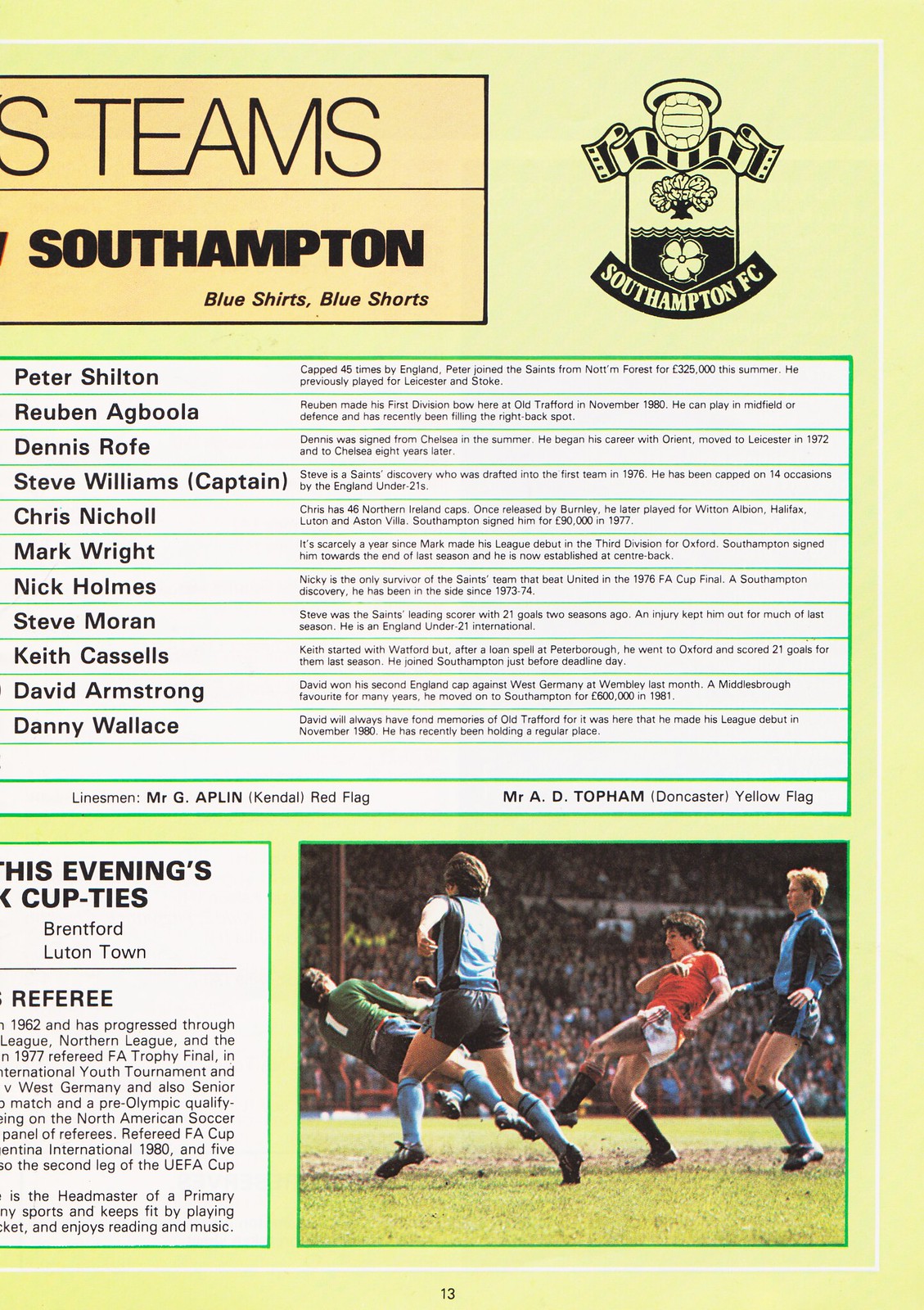The image appears to be the right half of a football program page, likely page 13 or 18, set against a pale yellow background. Dominating the top is the Southampton FC logo with text nearby stating "SEA Teams: Southampton, blue shirts, blue shorts" and "S Teams Southampton, blue shirts, blue shorts." Below the logo, there's a detailed roster on a white background with black text, separated by green lines, listing players such as Peter Shilton, Ruben Agboula, Dennis Rofe, Steve Williams (Captain), Chris Nickel, Mark Wright, Nick Holm, Steve Moran, Keith Kessels, David Arbshon, and Danny Wallace. Each player's name is accompanied by a brief description of their stats, origins, and contract details. To the lower right, a vibrant photograph captures the intense action on the football pitch with players in jerseys of different colors—blue, red, green—engaging dynamically with the ball amidst players possibly including captains or goalies. In the lower left corner, there's a small article regarding the evening's cup ties and discussions with the referee, flanked by descriptions of linesmen Mr. G Aplin Kendall (red flag) and Mr. A D Topman Doncaster (yellow flag).